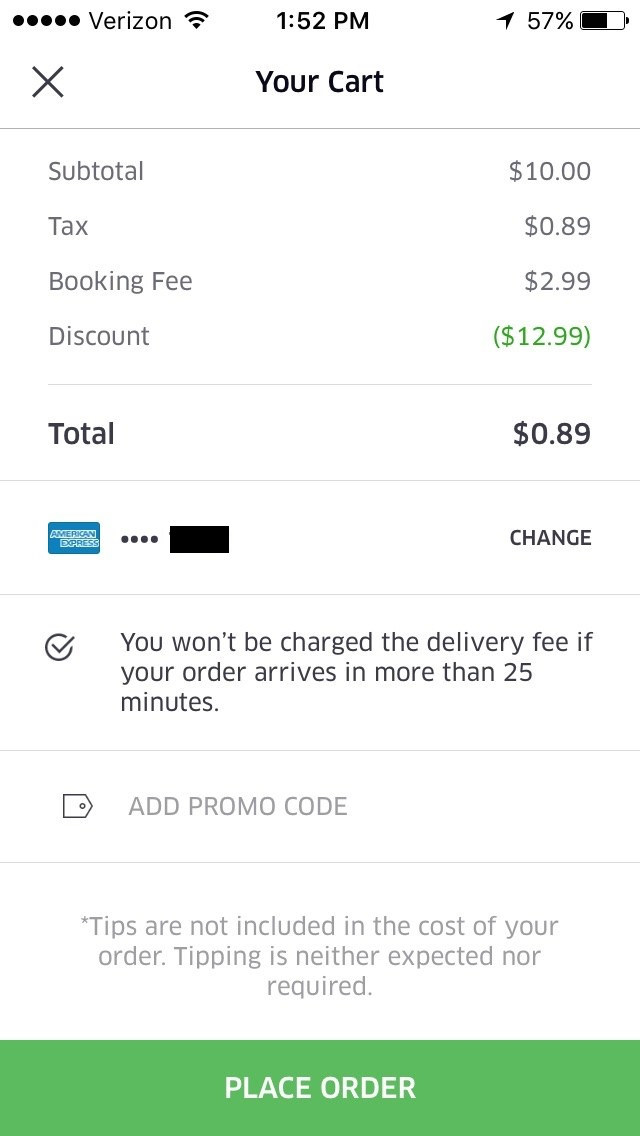A screenshot of a mobile shopping checkout screen displays various details on a white background. The user has Verizon with full signal strength, it's 1:52 p.m., and their phone battery is at 57%. The cart subtotal is $10, with an additional tax of $0.89 and a booking fee of $2.99. After applying a discount of $12.99, the total charge is reduced to $0.89, which is solely the tax amount since discounts can't be applied to it.

The payment method shown is an American Express card, with an option to change it indicated to the right. A checked circle informs the user that they won't be charged the delivery fee if the order takes more than 25 minutes to arrive. A section for adding promo codes is present, suggesting none have been applied. A note clarifies that tips are not included in the cost of the order, and tipping is neither expected nor required.

At the bottom, a prominent green box displays the option to "Place Order." The overall design is clean and straightforward, ensuring all necessary information is easily accessible for the user to finalize their purchase.